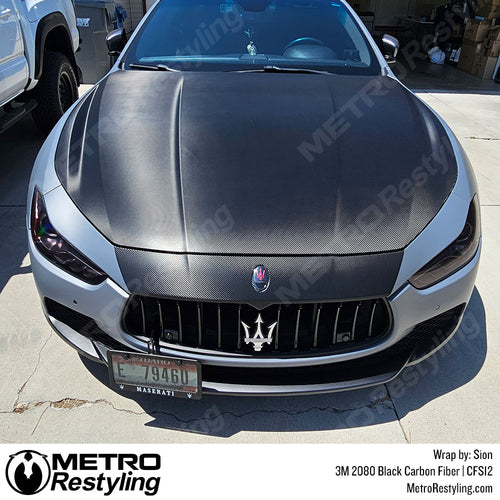The advertisement showcases a front-facing Maserati, prominently displaying its distinct badge with an arrow pointing up and two side arrows, sporting a fresh restyling and remodeling by Metro Restyling. The sleek vehicle features a light blue color on its sides with a striking 3M 2080 Black Carbon Fiber wrap on the hood and front grille. The Ohio license plate is clearly visible. The setting is a cracked concrete driveway, with a partial view of a white truck to the left. The image is branded with black lettering at the bottom: on the right, the Metro Restyling emblem and bold "Metro Restyling" text, and on the left, "Wrapped by Scion 3M 2080 Black Carbon Fiber CFS-12" along with the website "metrorestyling.com." A faint watermark of "Metro Restyling" covers most of the image subtly reinforcing the brand.